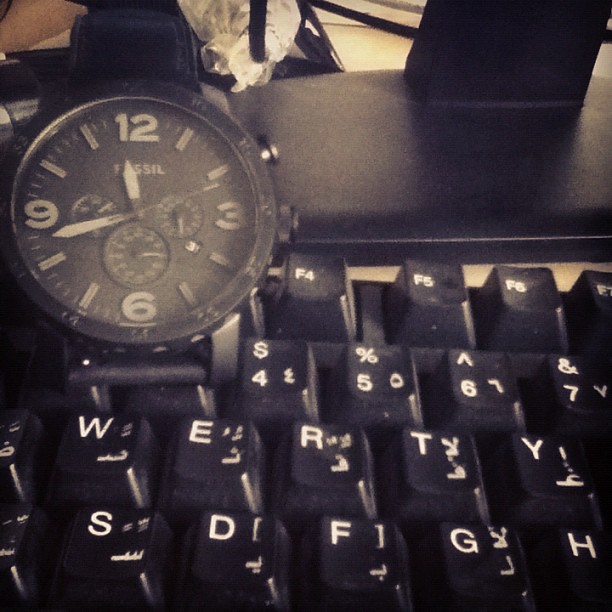In this black and white image, a sleek setup features a black keyboard and a sophisticated watch. The keyboard, with its white-printed black keys, is positioned in front of a computer monitor. Atop the keyboard rests a Fossil watch, its black band contrasting with the glass-covered black face. The watch showcases white Arabic numerals at 12, 3, and 6, with long white ticks marking other hours and four smaller ticks between each numeral. The brand name "Fossil" is visible just below the 12. Additionally, the watch face includes three smaller subdials, though their exact functions are obscured. The buttons on the side of the watch hint at timer functionality. The entire scene suggests a workspace, indicated by the partial view of the computer monitor and its base.